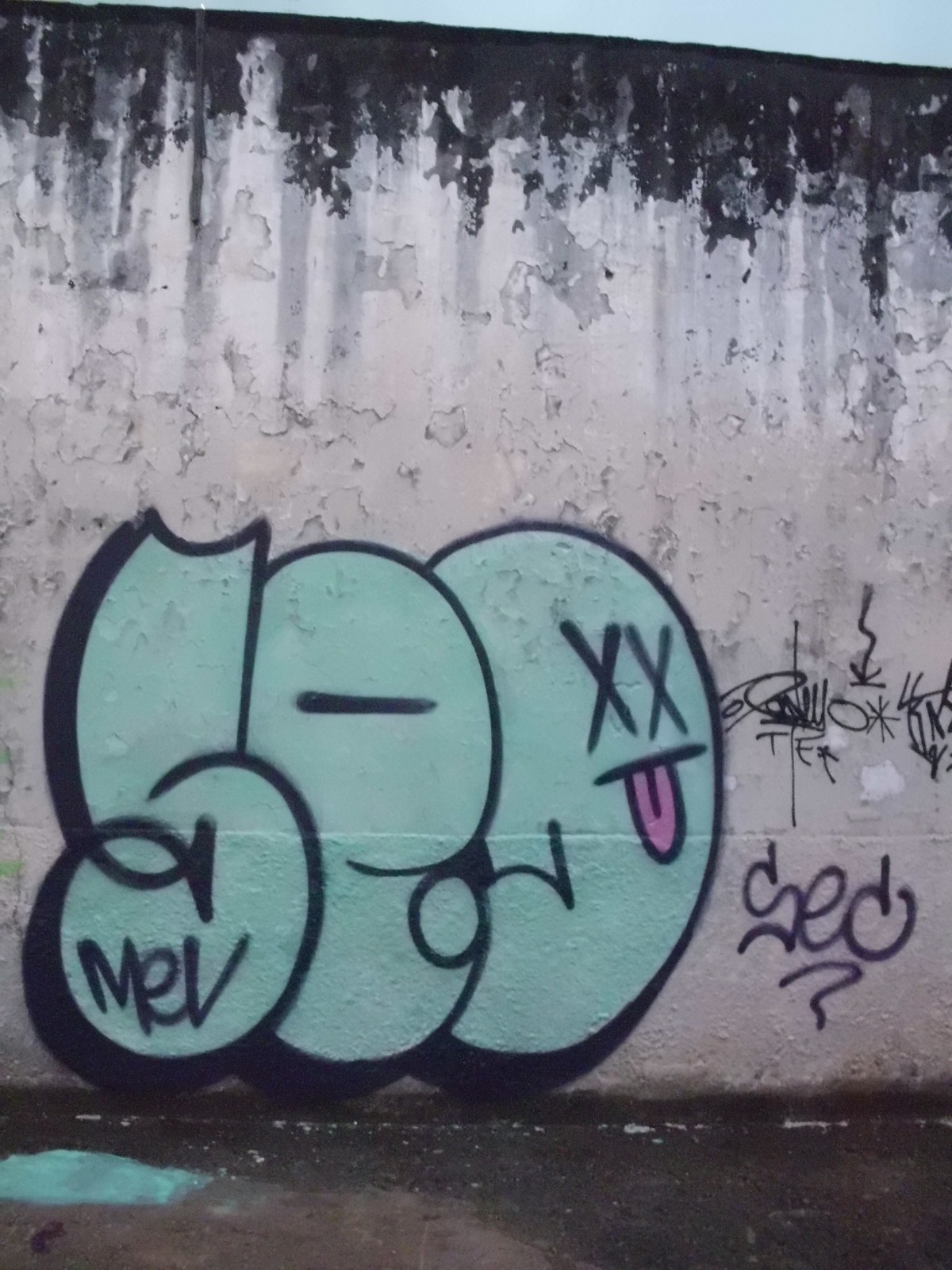The image is a color photograph in portrait orientation, showcasing a graffitied wall in a state of disrepair. The wall, primarily white, exhibits multiple layers of paint that are peeling, with remnants of black paint visible underneath. The graffiti is primarily blue-green, featuring stylized, graffiti-like elements. A notable part of the artwork includes a blob-like shape resembling a face, with X's for eyes and a protruding tongue. Adjacent to this face are large letters: S, E, and O, depicted in a baby blue hue. Below the 'S' are the capital letters "M-E-V," and near the 'E' the letters "S-E-C" can be seen, partially obscured by what appears to be a question mark and other black scribbles. The concrete floor below the wall has blue-green paint drippings, adding to the overall chaotic aesthetic of the scene. The image may capture the graffiti as a form of street art, potentially for documentation or admiration.